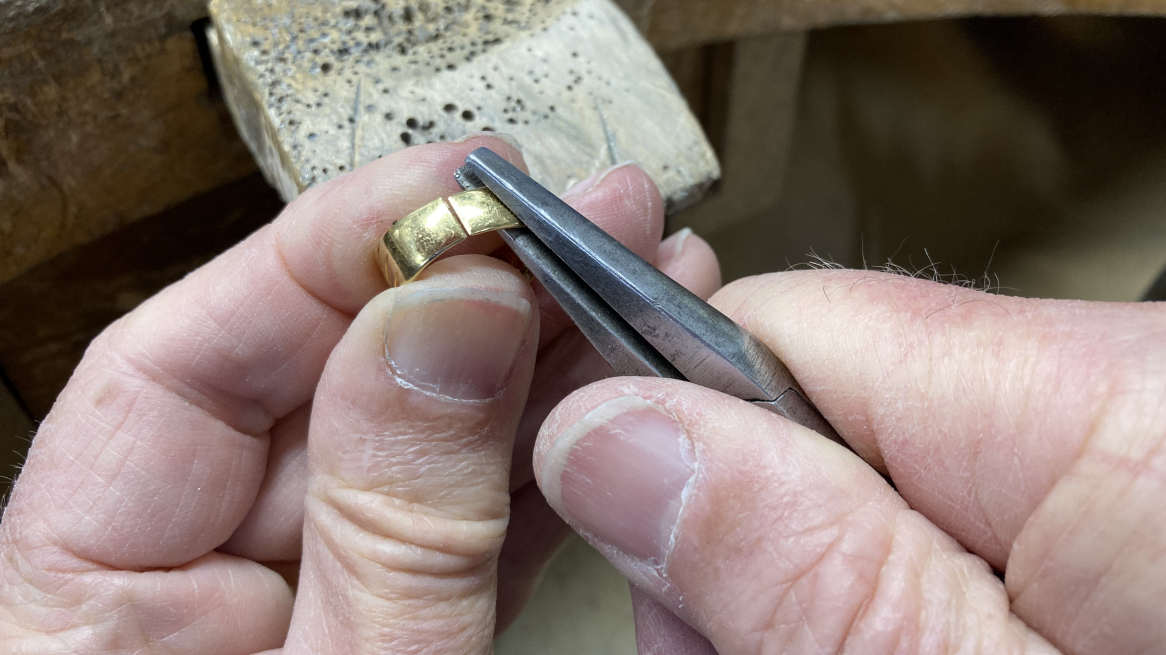In this detailed digital photograph, a close-up reveals a pair of dry, Caucasian hands working meticulously on a gold ring, underscoring the intricacies of the jeweler's craft. Emerging from the lower corners of the image, the left hand holds the gold band between the thumb and forefinger, while the right hand wields a silver, dark gray pair of pliers or a clamp close to the neck for enhanced control. The jeweler appears to be either resizing or repairing the ring, possibly removing a portion of soft, scratched gold. His hands rest on a large piece of stone, suggesting a sturdy surface for delicate work. The colors within the photo highlight shades of pink, gold, silver, and brown, creating a vivid representation of the jeweler's concentrated effort in connecting the ends of the gold ring together.